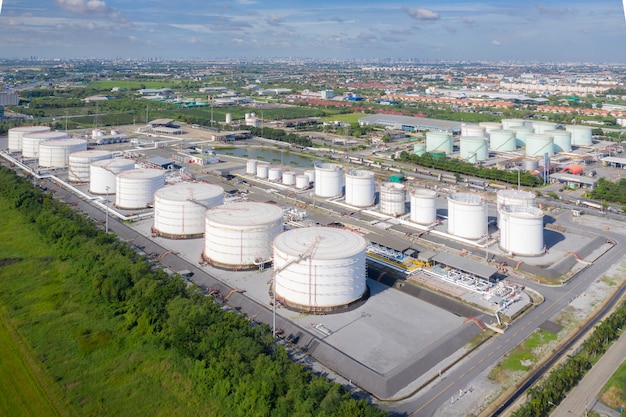This overhead photograph, likely taken from an airplane or helicopter, captures a sprawling industrial facility, possibly a water treatment plant, covering several miles of land area. Central to the image are multiple rows of large, cylindrical white tanks or silos, with the first row showing about nine such silos. These tanks seem to be designed for the functional storage and treatment of liquids, possibly water. Roadways are neatly laid out between each row of silos, promoting efficient access and oversight. In the background, similar green silos are visible, suggesting an extension of the same facility or a related industrial operation. The surrounding area is a mix of trimmed grass and wooded patches, adding a touch of greenery to the otherwise industrial landscape. The photograph is taken during the middle of the day, evident by the bright sunlight illuminating the entire scene. Additionally, beyond the facility, a city or townscape can be discerned, providing context to the facility's location.